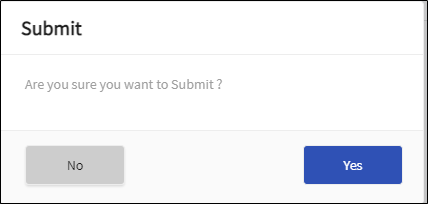This landscape-format image, captured in color, showcases a screenshot of a pop-up window against an undefined background, suggesting it was taken from a laptop or desktop computer due to its horizontal orientation. Dominantly white with a subtle black border around its edges, the pop-up window features a black "Submit" heading with a capital 'S' in the top left corner. Below this heading, a simple prompt reads, "Are you sure you want to submit?" with no accompanying text box. The interface offers two decision buttons: a gray "No" button on the left and a blue "Yes" button with white text on the bottom right, both designed for user interaction. The exact origin of the thin black border—whether inherent to the screenshot or added post-capture—remains uncertain.